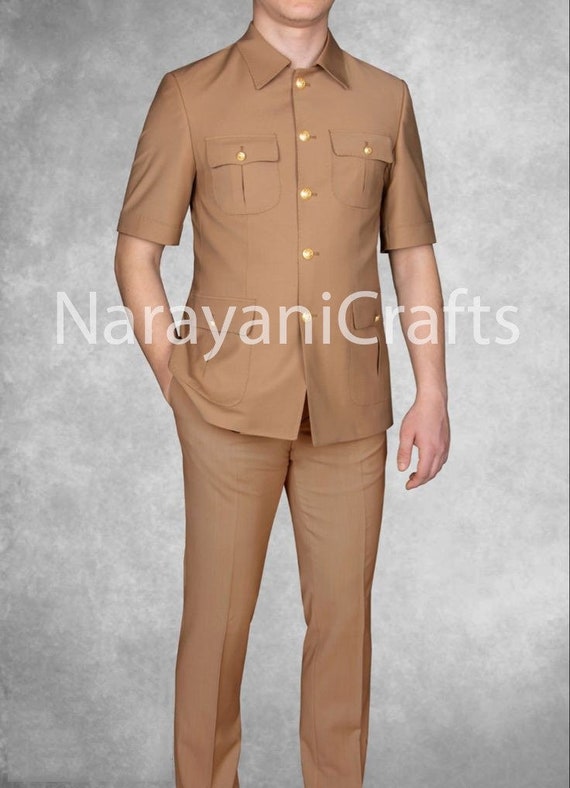A partially obscured man stands for a portrait, showcasing an outfit against a cloudy gray background, with only his chin visible. The outfit, seemingly crafted by Narayani Crafts—a name prominently watermarked at the center—exudes a casual yet refined style reminiscent of Western-influenced, Mao-era clothing with a military-like aesthetic. The ensemble is a uniform beige-brown color with a subtle sheen, suggesting a satin-like material. The untucked shirt, featuring a large collar and short sleeves, is adorned with gold buttons that run down the center and secure the four pockets—two on the chest and two at the hips. The matching straight, slim-fitting pants have a noticeable crease down the center. The man's right hand rests casually in his pocket, while his left hand hangs open by his waist, completing the poised yet relaxed stance.